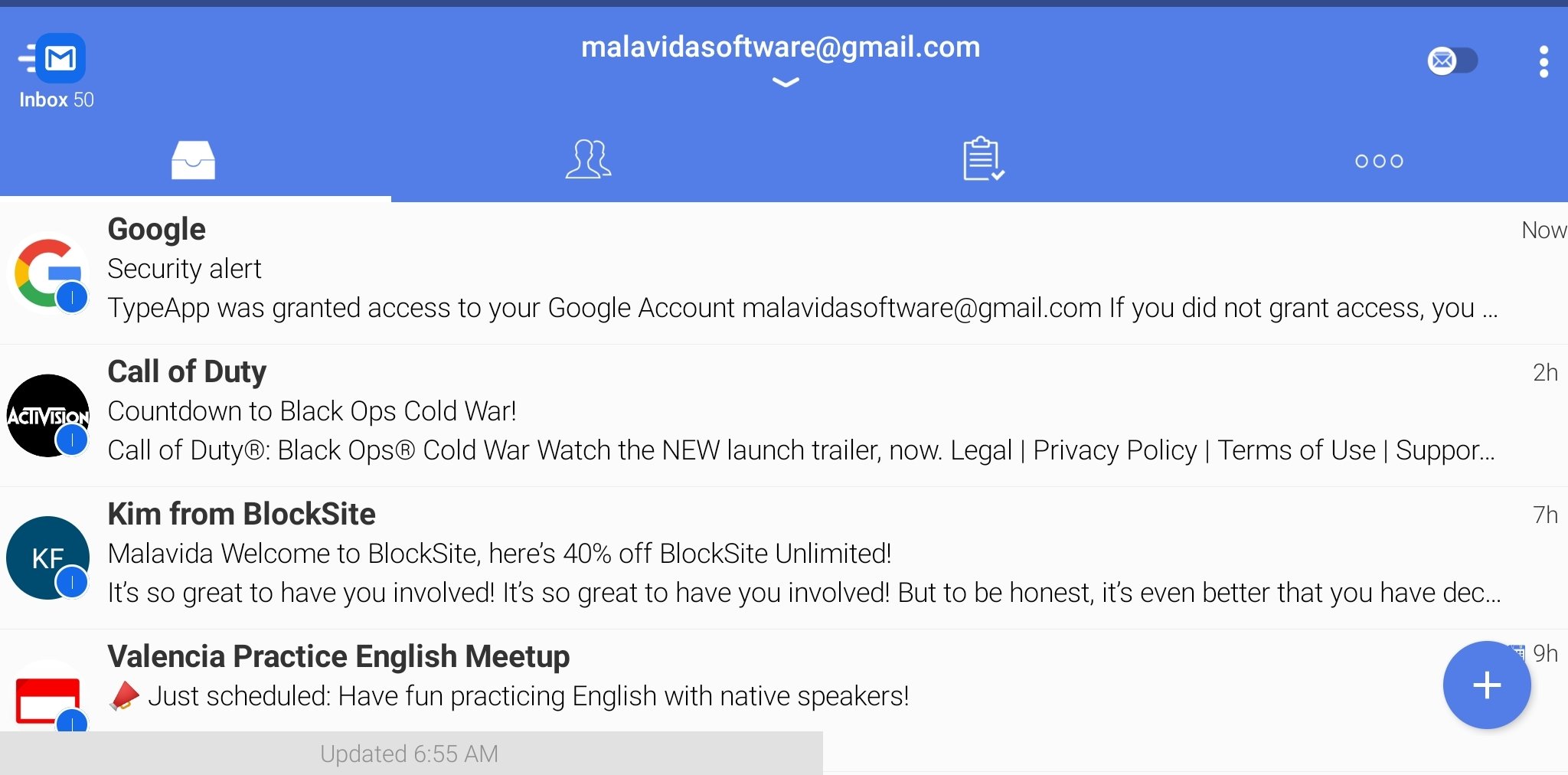This image showcases a website interface, focused around an email platform. The top section features an elegant dark blue header with the text "Malavida software at gmail.com" prominently displayed in white. Below this text, a downward arrow is visible. 

On the left side of the interface, there is a navigation panel that includes an "Inbox" label followed by the number 50, indicating the count of unread messages. Above this, there is a blue icon featuring a white "M". To the right of the navigation panel, a vertical slider and a trio of vertically aligned dots (menu icon) are present.

The main display area under the header contains various icons and notifications. These include a white file icon, images of people, a noteboard symbol, and a series of three horizontally aligned hollow dots. 

At the bottom section of the webpage, set against a gray background, a "Google security alert" message is displayed. This section contains a multicolored "G" logo (red, yellow, green, and blue), accompanied by a warning that reads: "Security Alert: Type Apple's granted access to your Google account Maldivas software at gmail.com. If you did not grant access, you…". The text is partially visible and appears to truncate.

Additional notifications and messages are visible in this section: 
- A "Call of Duty, countdown to Black Ops Cold War" banner, promoting a new trailer.
- A message from "Kim from Block Site" welcoming the user and offering a 40% discount on Block Site Unlimited.
- An update notification for "Valenicia practice English meetup" that reads: "Just scheduled have fun practicing English with native speakers. Updated at 6:55".

To the right side, a blue circle with a white plus sign within it is seen, likely indicating an option to add or create new content. Each category mentioned has its own icon positioned to its left for easy identification.